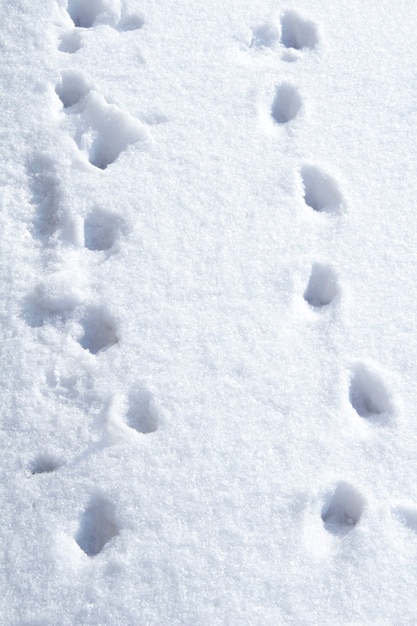This photograph captures the scene of fresh, white snow, fully illuminated by sunlight, creating a glossy and pristine backdrop. The snow appears dry and fluffy, typical of newly fallen snow, and it's quite deep, suggesting several inches of accumulation. Prominently featured in the image are two distinct rows of animal tracks, each consisting of small, slightly elongated, round or oval impressions that dig deeply into the snow. The right row comprises six prints, and the left row consists of seven prints, with the left side exhibiting some darker, shadowed areas and additional smudges—possibly indicating the presence of an animal dragging an appendage like a foot, arm, or tail. The tracks crisscross in a zigzag pattern from top to bottom, with a crisp, clear delineation on the right compared to the more disrupted left side, which has additional scuffed marks. Overall, the scene succinctly captures the intricate footprints against an untouched snow canvas, invoking a sense of mystery about the creatures that left these marks amidst an otherwise serene snowscape.